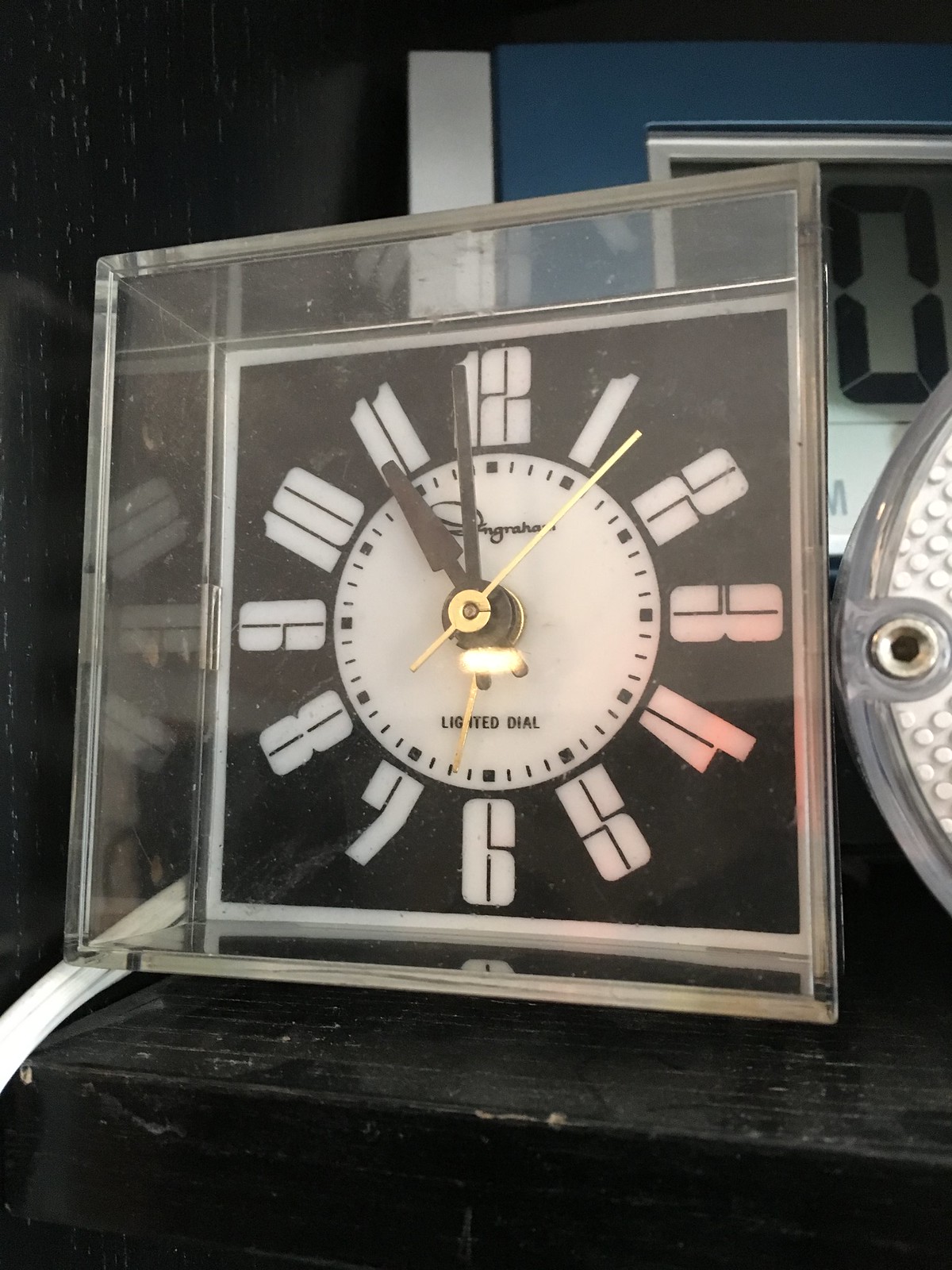The photograph showcases a clock encased in a clear, protective acrylic case. The clock has a traditional round face with a black background and bold, white numerals ranging from 1 to 12. The time displayed is 10:59, with the second hand positioned at 6 seconds. The clock's hour and minute hands are black, while the second hand is gold. At the top of the clock face, there's a signature or brand name, which appears to be "Syngram," though it is hard to read. Beneath this, the text "lighted dial" is visible at the bottom of the clock face. This clock is situated on a black, possibly wooden surface that shows some signs of aging and wear, with white lining details. To the right of the clock, the edge of another clock is just visible, and in the background, there is a flat, blue and white device with a prominent zero on its large LED display.